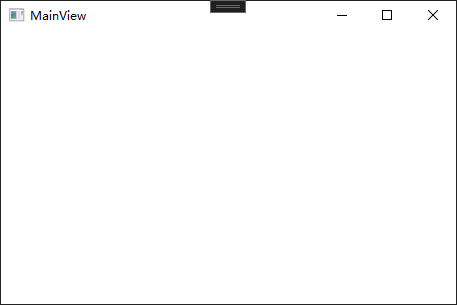The image is a screenshot from a website, framed by thin black lines on all four sides, forming a slightly wider-than-tall rectangle. In the upper left corner, the text "mainView" is displayed in gray font, with a capital 'V' in 'View'. To the left of this text, a small gray square contains a tiny left-aligned rectangle. At the top center, there is a tiny black rectangle, housing a very dark gray rectangle within it. On the upper right, there are standard browser window controls: a gray 'X' for closing the window, a gray outlined square for maximizing it, and a gray minus sign for minimizing it. The overall image provides a simple and minimalistic representation of a browser interface.